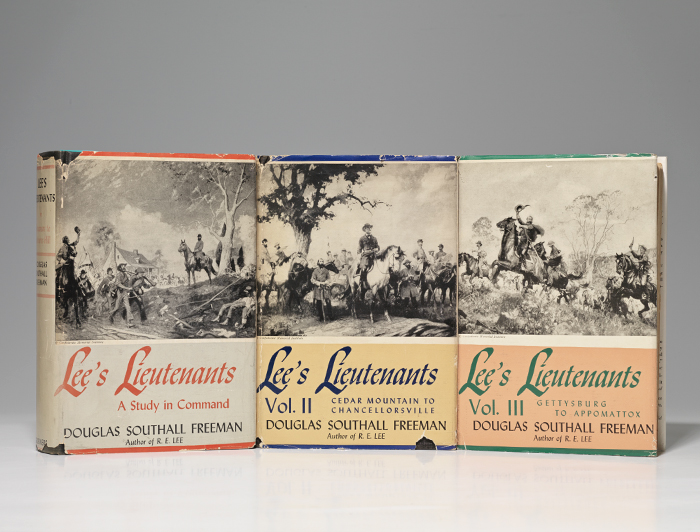The image showcases a professionally shot photo of three books titled "Lee's Lieutenants" by Douglas Southall Freeman. These volumes, focusing on the Civil War and 1800s United States history, are arranged upright against a gray background with a white countertop foreground. The first book, with an orange and white cover, is "Lee's Lieutenants: A Study in Command" and depicts a battle scene with men charging and a figure on horseback overseeing from a hill. The middle book, "Lee's Lieutenants, Volume 2: Cedar Mountain to Chancellorsville," features blue text on a yellow background with an illustration of a commander atop a white horse leading his officers. The final book, "Lee's Lieutenants, Volume 3: Gettysburg to Appomattox," has green text on a peach background and shows a commander charging on a battlefield. Together, they present a detailed visual and written exploration of key Civil War battles and leadership.